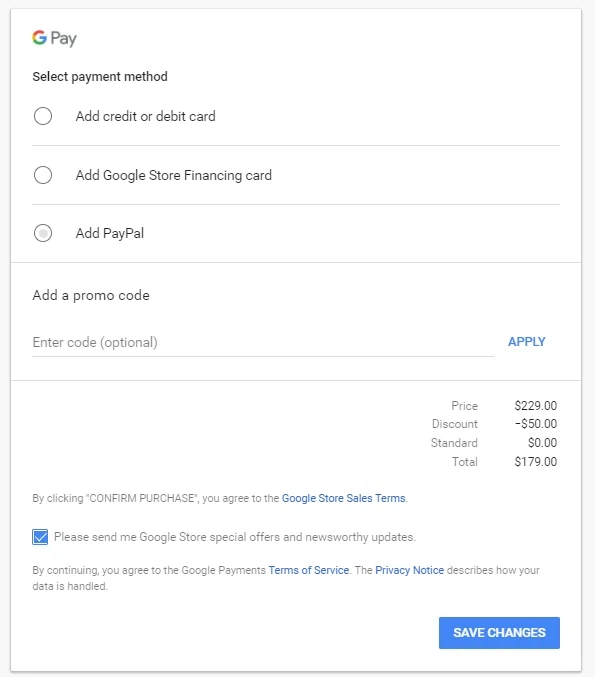Sure, here is a cleaned-up and detailed caption for the described image:

---

The image is a screenshot of a Google Pay checkout page. The interface presents a plain design with a white background and black text, separated by thin lines. The content is predominantly left-aligned. 

At the top-left corner, the Google Pay logo is displayed, featuring the iconic multicolored "G" in red, yellow, green, and blue next to the words "Google Pay." The page prompts the user to select a payment method, offering three radio button options:

1. Add credit or debit card
2. Add Google Store Financing Card
3. Add PayPal

In the screenshot, the user has selected the third option, "Add PayPal." Below these options, there is a section where users can enter a promo code, accompanied by a designated input line. The total amount due is prominently displayed at the bottom of the page, totaling $179.